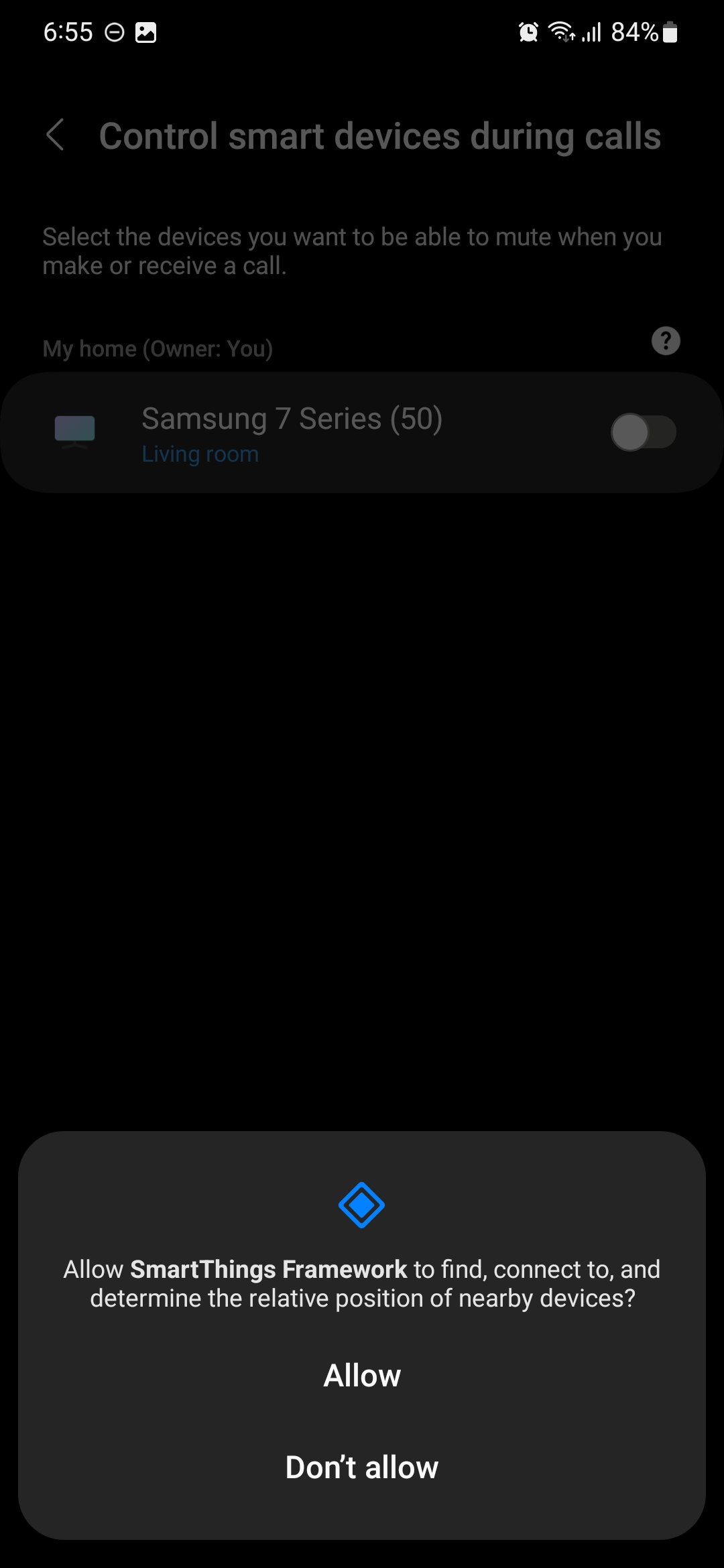A vertical screenshot of a mobile device with a jet black background. The time displayed at the top left corner is 6:55, accompanied by two icons. At the top right corner, there is an array of icons including an alarm, two Wi-Fi signals, and a battery icon showing 84%. Below this, translucent text reads: "Control smart devices during calls" with a left arrow icon next to it. Following that, it states, "Select the devices you want to be able to mute when you make or receive a call."

The main content lists under "My Home Owner You," with "Samsung 7 Series (50)" labeled next to it. Beneath this, in blue text, it says "Living Room." Adjacent to "Samsung 7 Series" is a toggle slider currently turned off and a question mark icon above it.

At the bottom, a dark gray pop-up box appears, featuring a blue diamond at the center. Above the diamond, it instructs, "Allow SmartThings Framework to find, connect to, and determine the relative position of nearby devices." Two clickable options, "Allow" and "Don't Allow," are displayed in bold white text at the bottom of the pop-up.